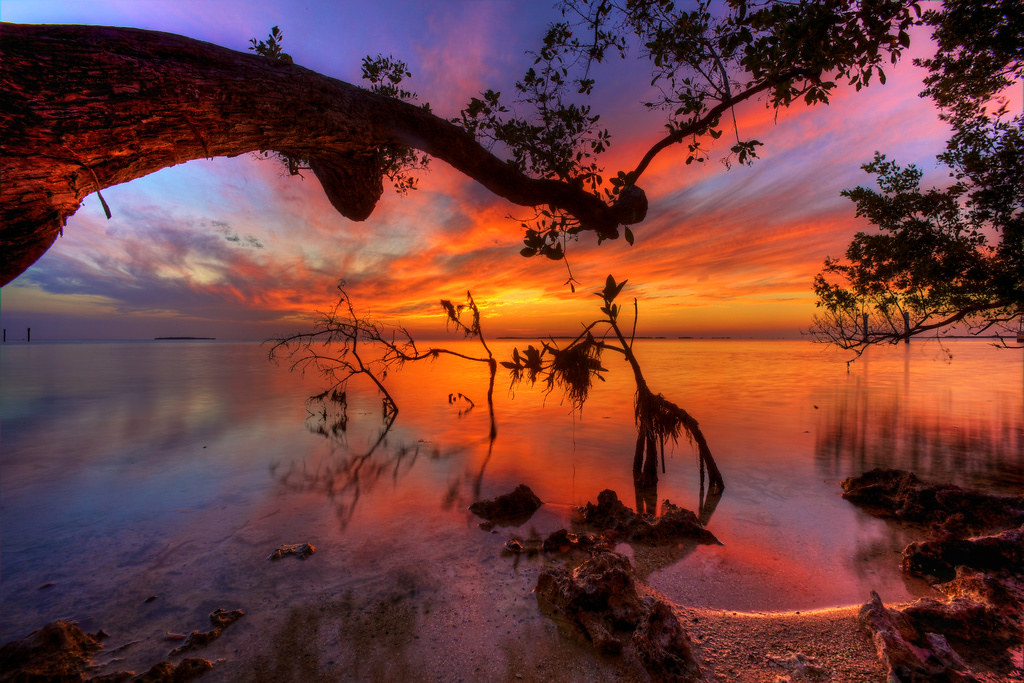The image captures a breathtaking sunset over a serene lake. The horizon, where sky meets water, is bathed in a mesmerizing palette of golds, oranges, purples, and blues, creating a warm and inviting hue. The sky is filled with billowy, white, and smoky clouds radiating towards the camera, their colors beautifully reflected on the lake’s surface. The left side of the water glows blue, transitioning to vivid oranges and yellows where the sun is hitting it, with hints of pink and purple blending in. In the foreground, a thick tree branch extends over the water, becoming silhouetted against the colorful sunset. Other branches and leaves are slightly visible, casting faint reflections in the water. The shoreline is barely visible, just a narrow, sandy strip at the image’s bottom. Overall, the scene is a harmonious blend of natural elements, creating an awe-inspiring and tranquil vista.